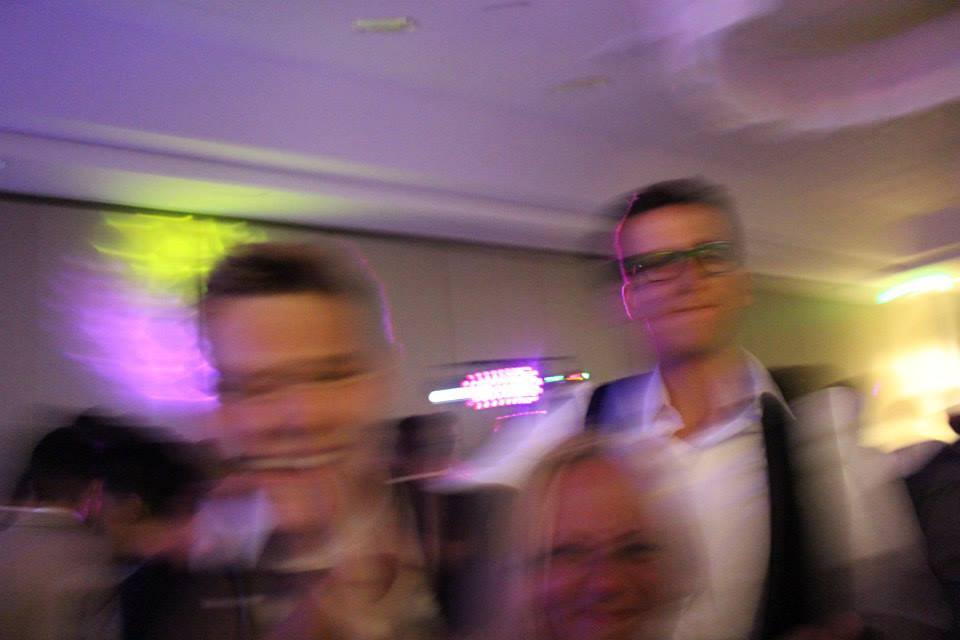In this blurred photo, four people are present. Three are facing the camera while one, on the far left, is only visible from behind, with dark brown or black hair in a ponytail held by a purplish scrunchie. The three facing the camera include two men and a woman positioned between them. The man on the left, who has short brown hair, is smiling broadly and is dressed in a black suit with a white collared shirt. The woman in the center sports blonde hair and glasses, smiling warmly with her nose scrunched up, but not showing her teeth. She is partially obscuring the second man on the right, who also has short hair and is wearing glasses with possibly green or blue frames. He is dressed in a white button-down shirt with a black vest and is not smiling as broadly as the others. The background features a cream-colored wall with a white ceiling and is illuminated by various neon and bright lights, including green, pink, purple, and yellow hues. These lights emanate from wall signs and create a lively, party-like atmosphere, although the overall image remains moderately lit, suggesting the main lights might be dimmed.